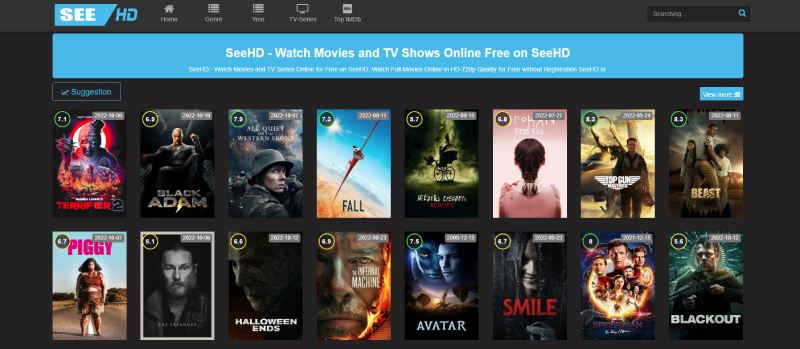This image is a screenshot from a website featuring a dark charcoal gray background. At the top, a lighter gray horizontal rectangle spans across, creating a header. On the left side of this header, there's a diagonally cut blue rectangle with the white text "SEE". Adjacent to it, the abbreviation "HD" is displayed in blue font, followed by menu items labeled "Home", "Genre", "Year", "TV Series", and "Top IMDB", all in white. Towards the far right side, there is a search field with the placeholder text "Searching..." in gray, accompanied by a gray magnifying glass icon.

Below the header, a prominent blue banner contains the white text "CHD - Watch Movies and TV Shows Online Free on CHD". Beneath this, another line of smaller white text is present, though it is too low quality to read clearly. Further down, a small blue button with the word "Suggestions" in white font can be seen. Lastly, the screenshot showcases two rows displaying various movie cover art, reminiscent of traditional movie box covers.